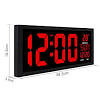This image depicts a grainy representation of a flat, digital alarm clock, potentially an advertisement or low-resolution computer clip art. The clock, angled to appear three-dimensional, features a prominent black background contrasted by bright red font displaying the time as "12:00". The numbers are large and central, with smaller, unreadable red and white text to the right. There are also faint grey arrows surrounding the clock, indicating dimensions or measurements. The white base provides a stark contrast to the predominantly black and red color scheme.